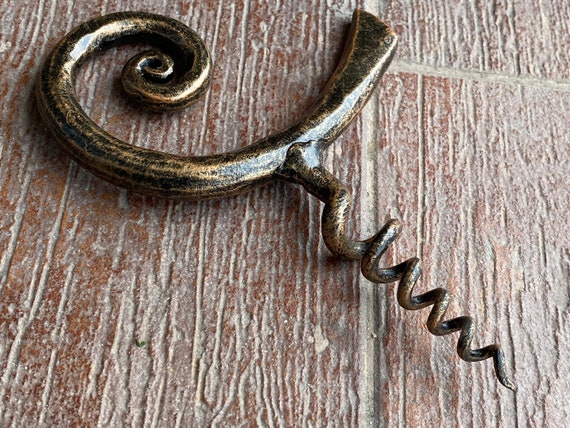This photograph captures a close-up of an ornate brass wine corkscrew displayed on a polished brown wooden surface. The corkscrew features an intricate design with a swirled handle, resembling a curved horn or antler, that curls tightly into a small centered circle. The metallic body of the corkscrew boasts a burnished gold and black finish, creating a striking shiny appearance. The spiral point of the corkscrew extends from the tight curl of the handle. The wine opener is positioned diagonally across the frame, and its detailed craftsmanship is highlighted by the light reflecting off its polished surface. The brown wooden table beneath provides a rich, warm contrast to the elegant corkscrew, which stands out as both a functional tool and a piece of art.